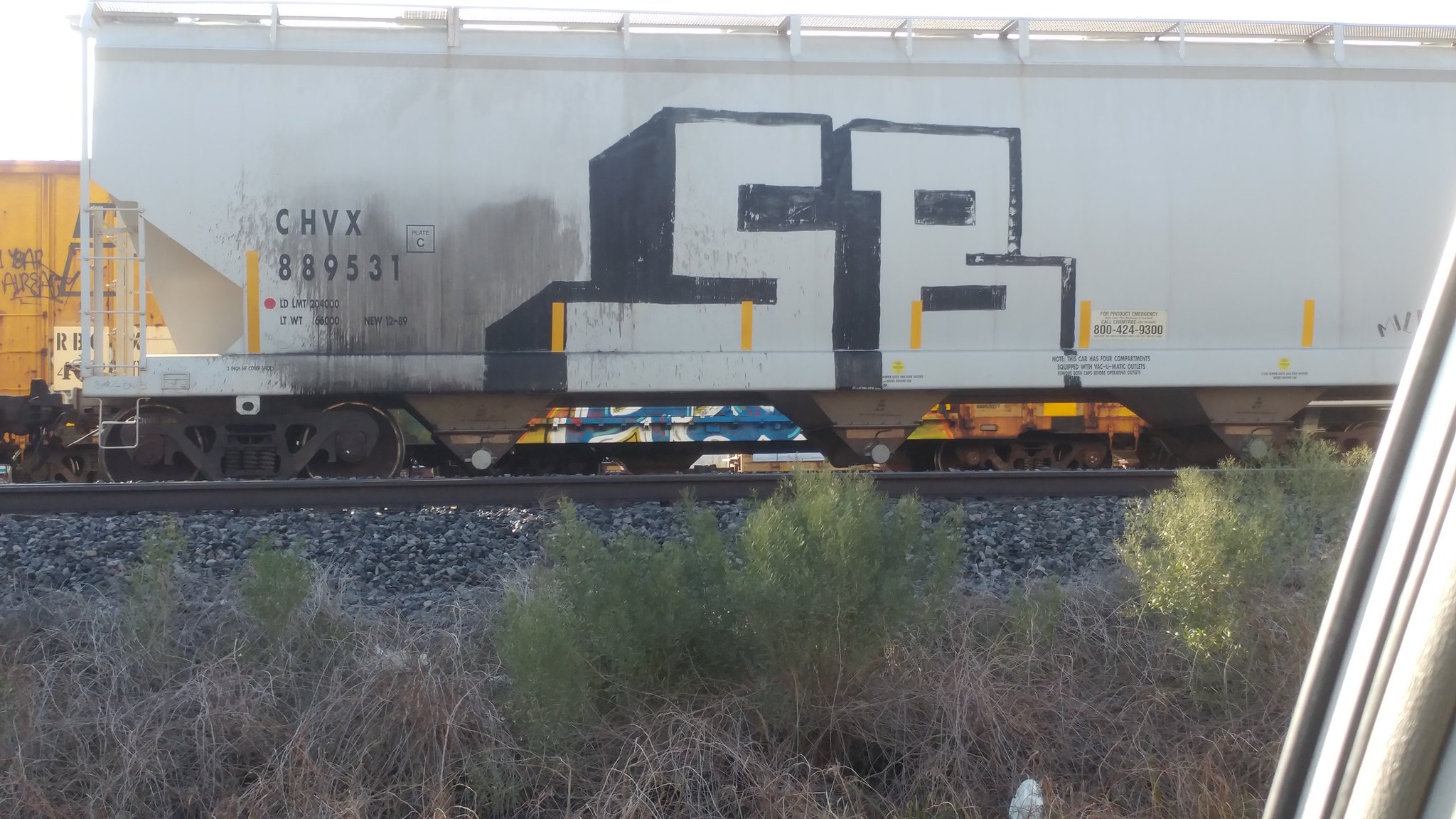The photograph captures a detailed scene of a train car, taken from inside a vehicle, with part of the car window visible on the right-hand side. The train car, predominantly light gray or white, features prominent graffiti in black block letters spelling "SB" or possibly "5B." It is notably marked with the letters "CHVX" and the number "889531" in black text on the left-hand side. The car is adorned with multiple vertical yellow lines, six in total, evenly spaced along its length. To the left of this train car, another yellow train car is partially visible, also covered in graffiti that is difficult to decipher. The scene takes place on brown train tracks surrounded by gravel and green shrubbery mixed with some beige-tan grass-like debris. Additionally, glimpses of a blue and yellow train car are visible behind the other train cars. The overall setting is bright and sunny, with the light source coming from the upper left, illuminating the entire scene without any clouds in sight.